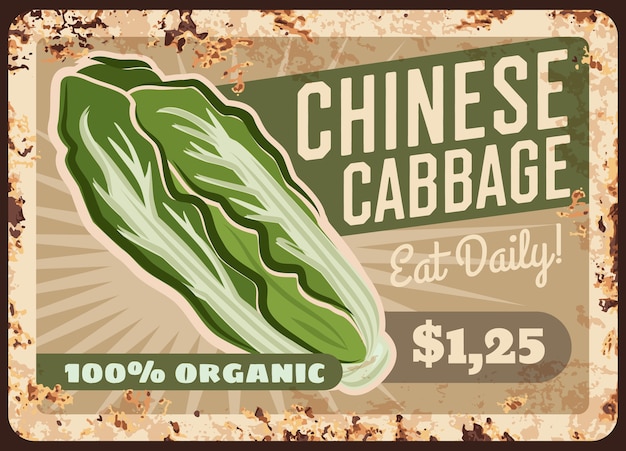The digital image portrays a vintage-style advertisement sign with a distressed appearance, echoing an old metal sign from the 1920s through the 1940s, possibly inspired by a style seen in Fortnite. The sign features a large, animated picture of Chinese cabbage in the center, with rays emanating from it as if highlighting its importance. The background is a light tan, heavily rusted and oxidized, with visible cracks and scratches that enhance its aged look. Surrounding the image is a dark brown border that frames the entire sign.

Prominent text on the sign reads "Chinese Cabbage" in white, capital letters, set against a green rectangle. Below it, “eat daily” is written in cursive, and the price “$1,25” indicates a foreign origin due to the comma in place of a decimal. The bottom of the sign declares “100% organic” in a light blue color, contrasting against the mainly light beige lettering of the other words. Overall, this sign effectively mimics the look of an antique advertisement with a blend of old-world charm and digital artistry.